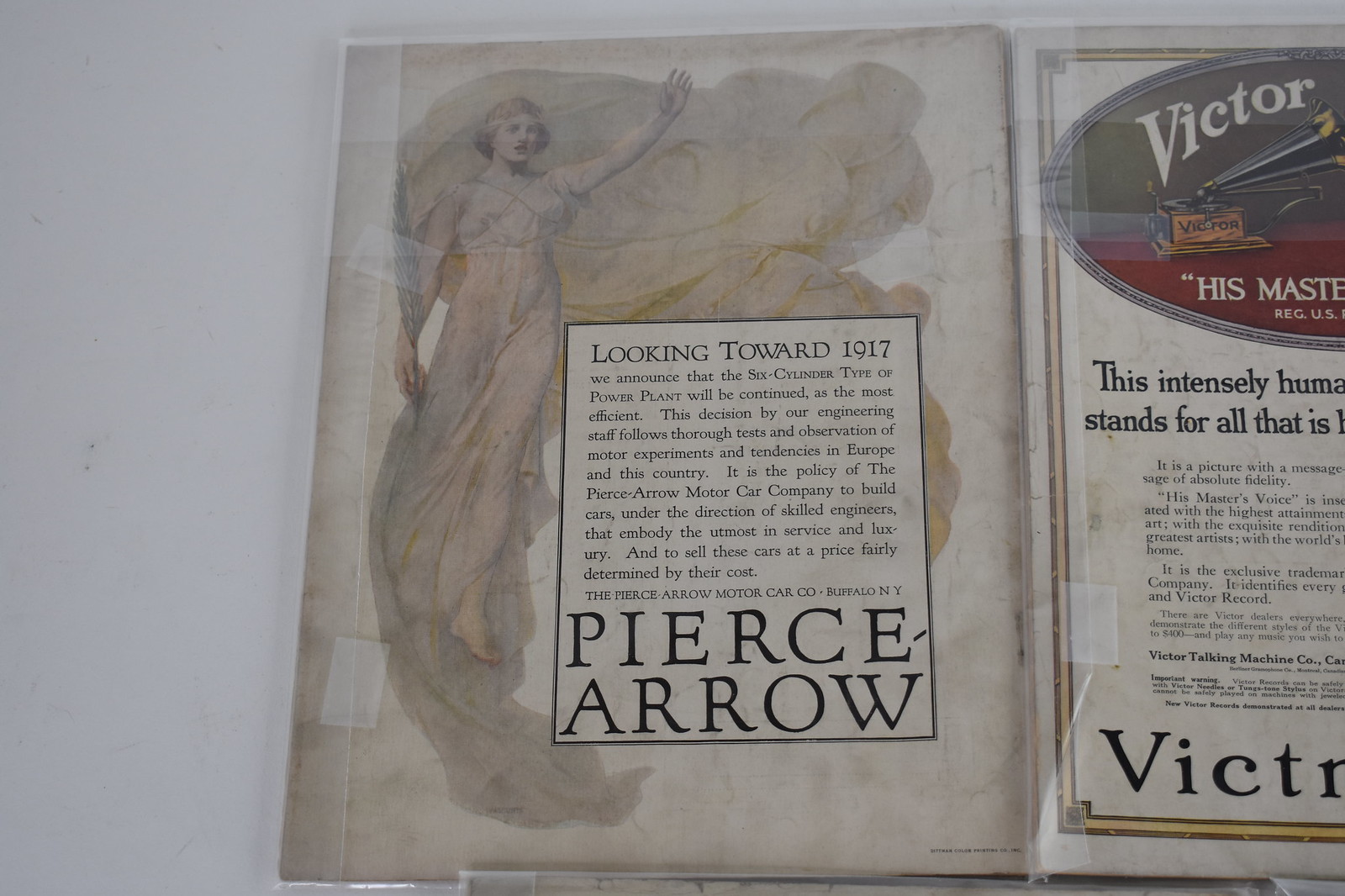This image displays an open white book with a split overview of its back and front covers. The left panel showcases the book's back cover, featuring an angelic woman dressed in white with yellow accents on the ends of her dress. She is holding a long white flower and has her hand raised. Accompanying her image is a block of text. The text reads: "Looking towards 1917, we announce that the six-cylinder type of power plant will be continued as the most efficient. This decision by our engineering staff follows through tests and observation of motor experiments and tendencies in Europe and this country. It is the policy of the Pierce Arrow Motor Car Company to build cars under the direction of skilled engineers and embody the utmost in service and luxury and to sell these cars at a fairly price fairly determined by their cost." The caption also mentions "Pierce Arrow."

On the right panel, the front cover of the book, a partial view of a sign that reads "Victor" at the top is visible. The sign appears to be a promotion for the Victor gramophones, with a phrase like "Victor is Master" and an illustration of a Victrola. However, the description is cut off, making it difficult to read the entire content. The page is adorned with green and red elements, and the text is enclosed within a yellow square. The lettering throughout the book is black and notably small, contributing to the difficulty in deciphering the complete details.